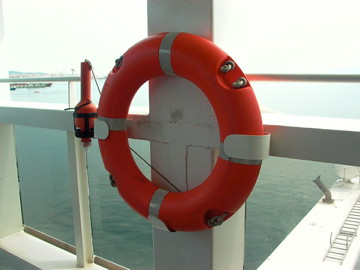This detailed photograph captures an orange life preserver ring securely fastened to a white railing aboard a ship. The lifesaving device, harnessed with a white clasp, is prominently placed against one of the railing posts. The railing features glass panes between its spokes, offering a clear view of the vast blue ocean beyond. The scene, likely taken during the daytime, shows the ship either docked or in motion across the water. Through the glass, additional details such as another bay and a distant boat are visible, enriching the marine backdrop. The image, set on what appears to be the second level of the ship, emphasizes the lifebuoy's readiness for use, encapsulating a serene yet practical maritime moment.